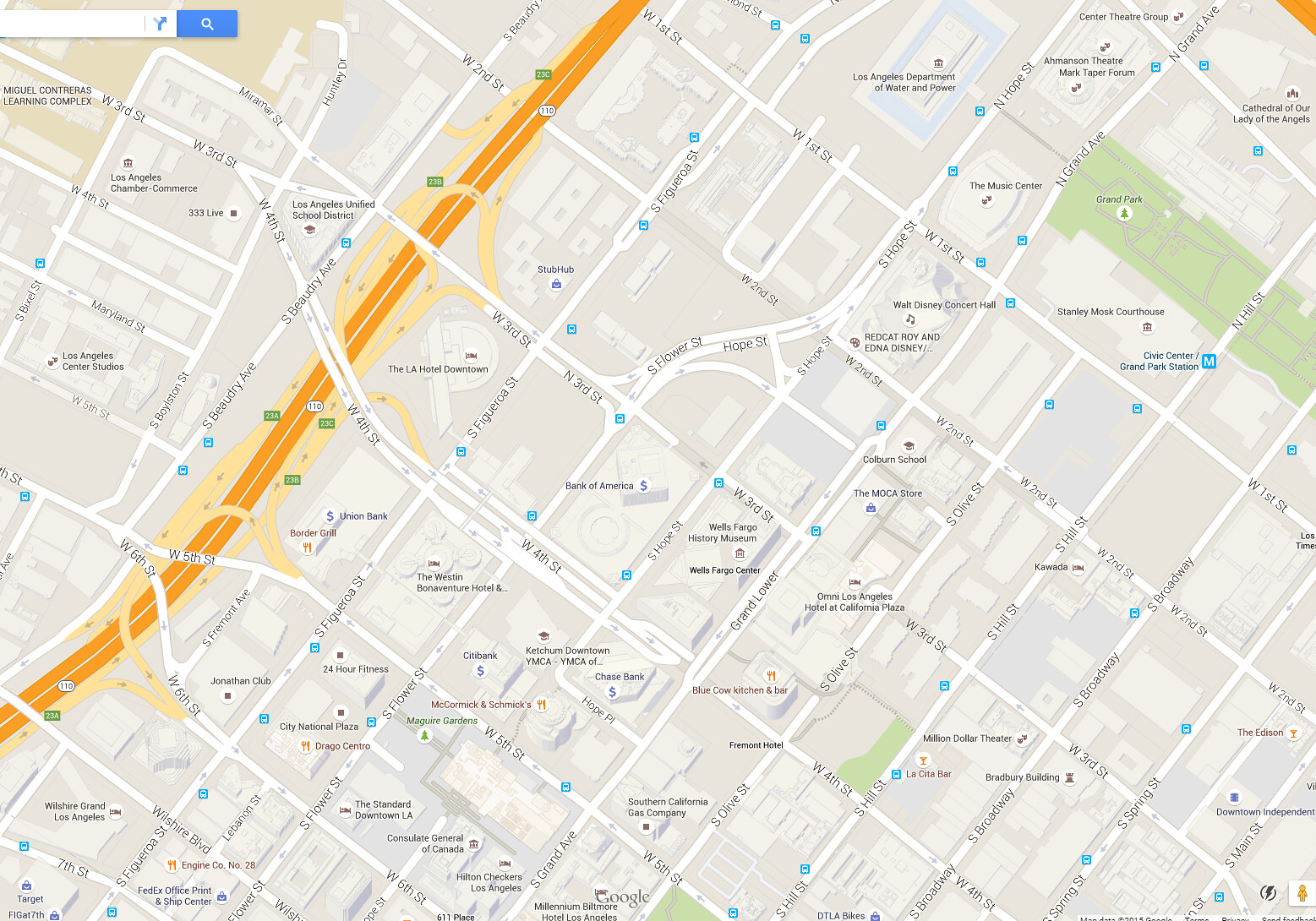This is a screenshot from Google Maps displaying a detailed, zoomed-out view of downtown Los Angeles. The map highlights various buildings and streets of the area. In the upper left corner, there is an empty, white search box with a small arrow to its right and a blue box featuring a white magnifying glass next to it.

Prominent locations pinpointed on the map include significant landmarks and institutions. Notable places such as the Los Angeles Unified School District, Wells Fargo History Museum, Wells Fargo Center, Bank of America, Civic Center, and Grand Park Station are visible. The map also highlights cultural and historical sites like the Stanley Mosk Courthouse, Walt Disney Concert Hall, Million Dollar Theater, and Bradbury Building.

Entertainment and hospitality venues like La Cita Bar, Blue Cow Kitchen and Bar, Fremont Hotel, Southern California Gas Company, the Westin Bonaventure Hotel, Union Bank, Border Grill, Jonathan Club, City National Plaza, and 24 Hour Fitness are clearly marked. Additionally, business and service places such as FedEx Office Print and Ship Center, Hilton Checkers Los Angeles, Consulate General of Canada, the Standard Downtown LA, Millennium Biltmore Hotel Los Angeles, DTLA Bikes, the Edison, and Redcat Roy and Edna Disney are identified, showcasing the vibrant and diverse infrastructure of downtown Los Angeles.